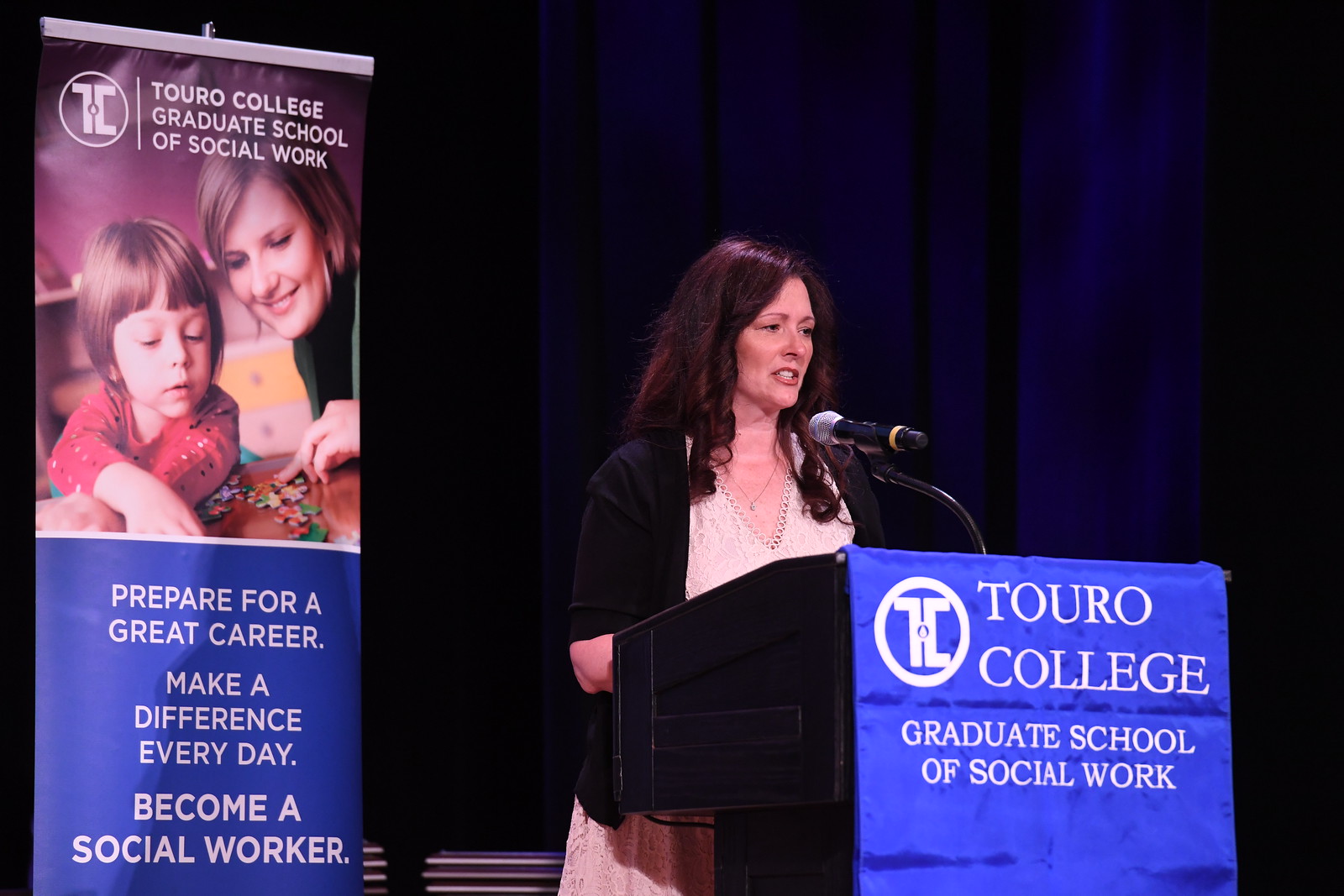The photograph captures a woman with brown, shoulder-length hair, mid-sentence, speaking into a microphone at a black podium. She is wearing a white blouse or dress with a black jacket, standing slightly to the right of the camera. The podium features a blue banner with white text reading "Truro College Graduate School of Social Work," accompanied by a circular logo with the letters "TC" in the center. Behind her, dark blue or purple drapes form the backdrop. To the left, a poster also for Truro College Graduate School of Social Work displays an image of a woman helping a young boy with a puzzle, with a caption beneath that reads, "Prepare for a great career. Make a difference every day. Become a social worker."